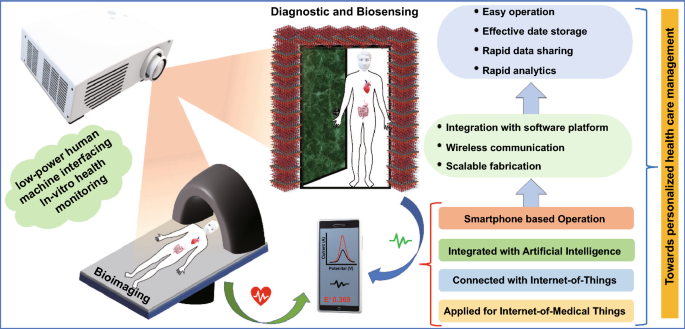This detailed illustration, reminiscent of a textbook diagram, portrays various advanced medical technologies for health monitoring and diagnostics. Starting in the upper left corner, we see a white machine featuring a knob and side vents. The label beneath it reads "Low Power Human Machine Interfacing in Vitro Health Monitoring." Directly below, an MRI-like setup is depicted, showing a gray table with an outlined, unclothed human figure lying flat, labeled "Bioimaging."

To the right, a chart resembling a heart monitor display is shown, characterized by a sequence of rising and falling peaks resembling a volcanic shape. In the upper center of the image, a man stands within a stand-up x-ray machine for a diagnostic test. The man, shown in a frontal view with arms at his sides, stands against a green backdrop. This section is labeled "Diagnostic and Biosensing."

Along the right side of the image, a vertical list highlights the system’s key advantages: "Easy Operation," "Effective Data Storage," "Rapid Data Sharing," and "Rapid Analytics." This comprehensive diagram encapsulates cutting-edge technologies and their applications in health monitoring and diagnostics.